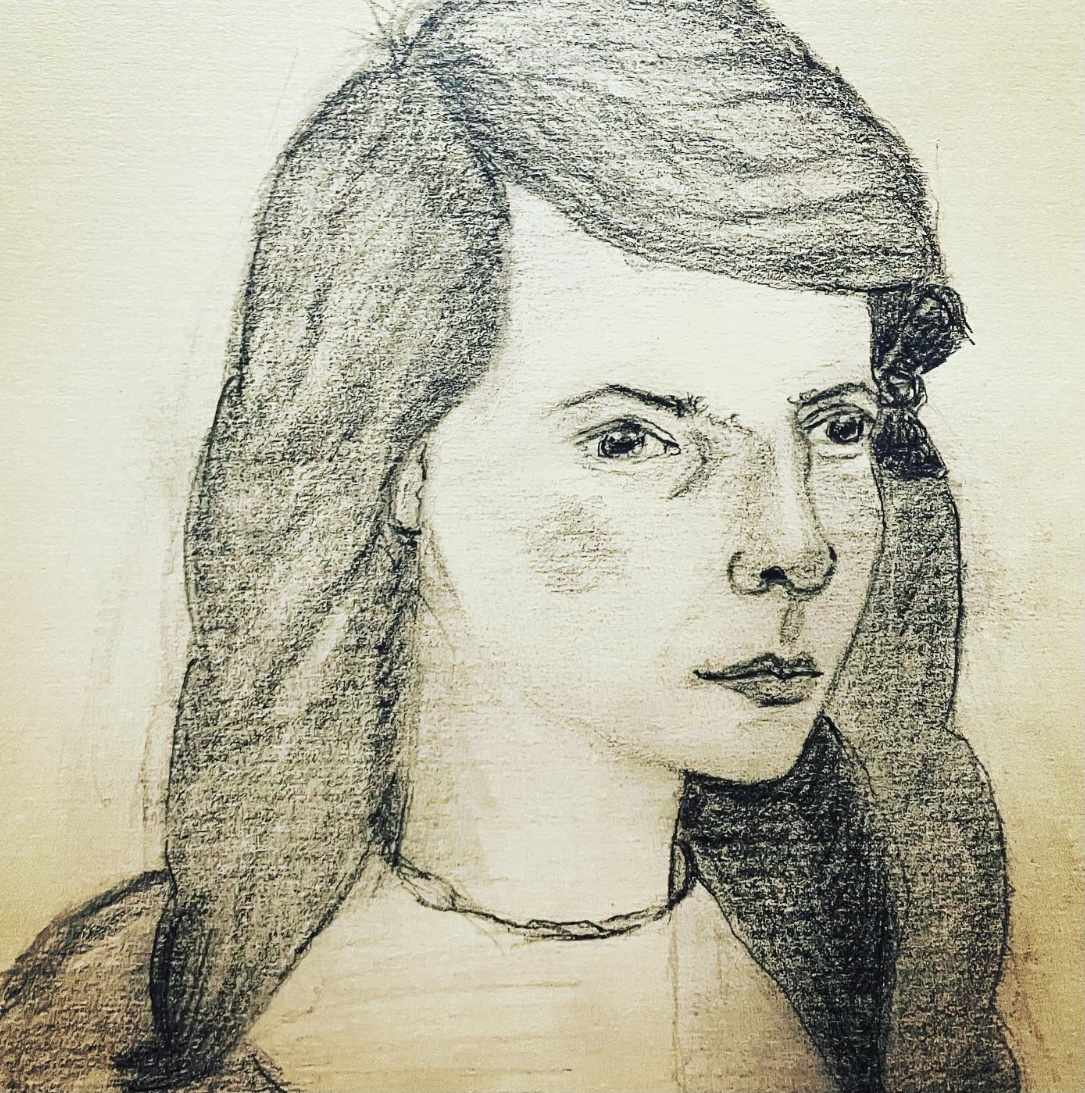The image shows an intricately detailed, realistic pencil sketch of a young woman, drawn on slightly gradient brown paper, transitioning from deep brown at the bottom to a creamy color at the top. The woman is looking to the right of the viewer, her expression serious and somewhat upset. She has long, flowing dark hair that reaches below her shoulders, parted at the side, elegantly framing her face and splitting into two bangs near her forehead. Her thin eyebrows arch delicately above her eyes, which appear slightly misaligned, giving a peculiar gaze. The woman has a narrow upper bridge of the nose and a small, pointed chin. Her lips are prominently accentuated with lipstick. She is adorned with a tightly wrapped necklace around her neck and is wearing a dress that is dark around the sleeves with a white, slightly ruffled collar, extending down the front. The shading in the drawing skillfully highlights the texture of her hair and the contours of her facial features, capturing the play of light and shadow with remarkable precision.